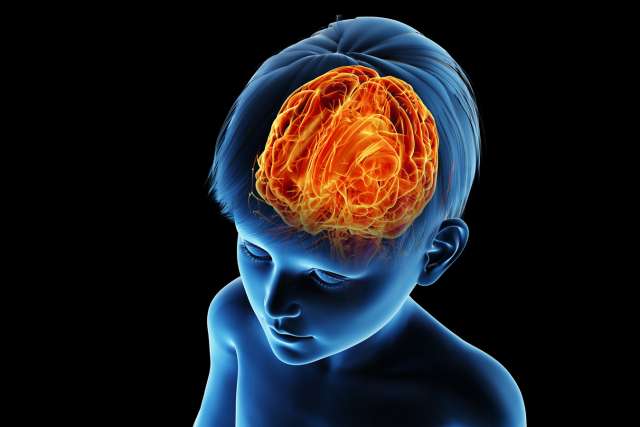In this horizontally rectangular digital artwork set against a stark black background, a computer-generated image of a young boy is prominently featured. The boy, rendered in an unnatural bluish hue, appears to be facing slightly to the left. His hair is short, cut above his ears, with some bangs falling forward. His eyes are closed, giving him a blank expression, and he's not wearing a shirt, with the image cutting off just below his shoulders, exposing only his upper torso.

The most striking feature of this piece is the depiction of the boy's brain, visible through his seemingly translucent skull and hair. The brain is illuminated in vivid shades of orange, yellow, and red, resembling fire more than a typical anatomical brain. This fiery brain, which maintains a general brain-like shape but is filled with swirling lines and squiggles, draws immediate attention and serves as the central focus of the image.